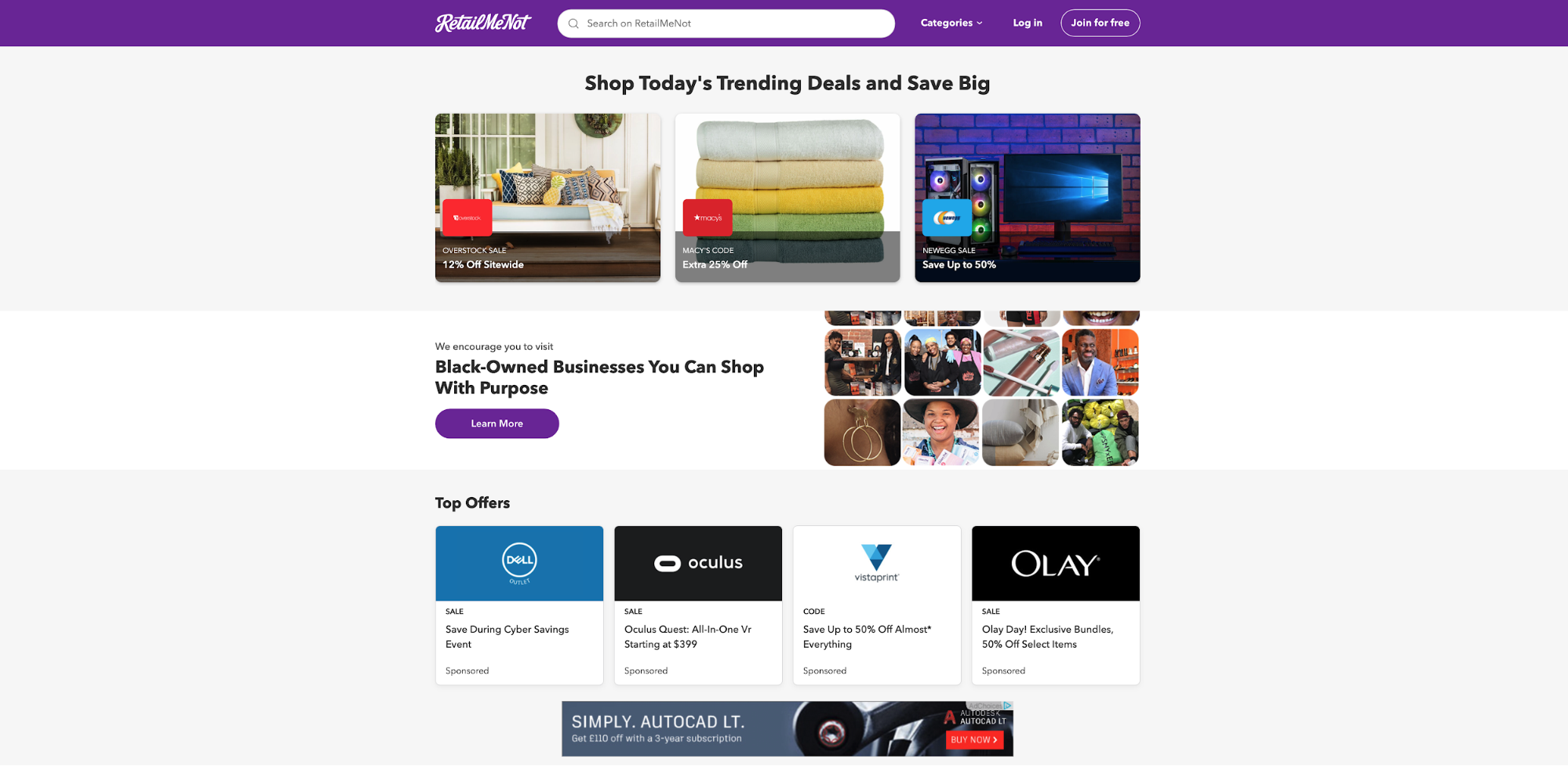The image is a screenshot from the RetailMeNot website. The top bar features a distinctive purple color with the site's name, "RetailMeNot," prominently displayed. Adjacent to this title is a search bar and a drop-down button labeled "Categories." To the right, there are options to "Login" and "Join For Free."

Below the top bar, a banner proclaims "Shop Today's Trending Deals and Save Big." Underneath this banner, there are three clickable photographs: the left image depicts a couch, the center image shows a stack of folded towels, and the right image appears to be an advertisement, potentially for a computer or speakers, though it is not entirely clear.

Following this, there is a section titled "Black Owned Businesses You Can Shop With Purpose," accompanied by a "Learn More" button and a series of thumbnail images. Further down, the "Top Offers" section features clickable logos for Dell, Oculus, an unreadable third logo, and Olay.

At the bottom, there is an advertisement for AutoCAD LT, marked by a noticeable red button in the bottom right-hand corner of its rectangle. The webpage's background varies in color: the top and bottom rows are light gray, while the middle section maintains a white background.